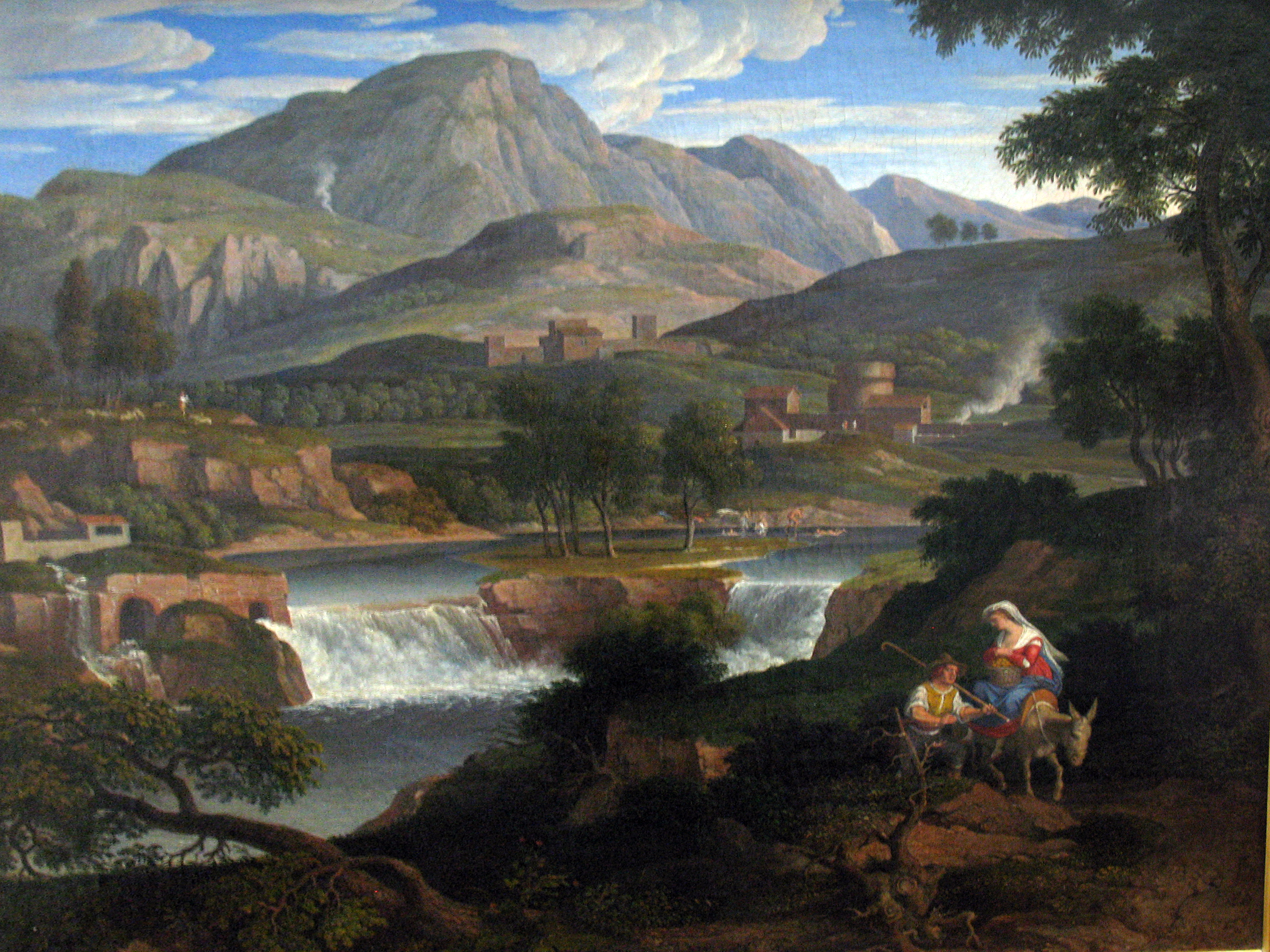The painting depicts a picturesque and expansive outdoor landscape brimming with details. Dominated by majestic mountains in the background, the scene features a bright blue sky adorned with big puffy clouds. The mountains transition into rolling green hills, speckled with rocky outcroppings and scattered trees. Nestled among these hills are various homes, including a distinctive farmhouse. 

A tranquil river flows from the right to the center, culminating in a fast-crashing waterfall before continuing downstream. The foreground showcases a woman seated on a donkey, adorned in a red long dress, a white veil, and a blue apron. Beside her stands a man, holding a staff. They are positioned along the edge of the riverbank, adding a human element to the serene landscape. Trees frame the corners of the painting, and a small building is nestled in the middle left. The overall scene is a meticulously painted portrayal of nature, enhanced by the vibrant colors of blues, whites, greens, reds, yellows, browns, and grays, creating a harmonious and detailed composition.